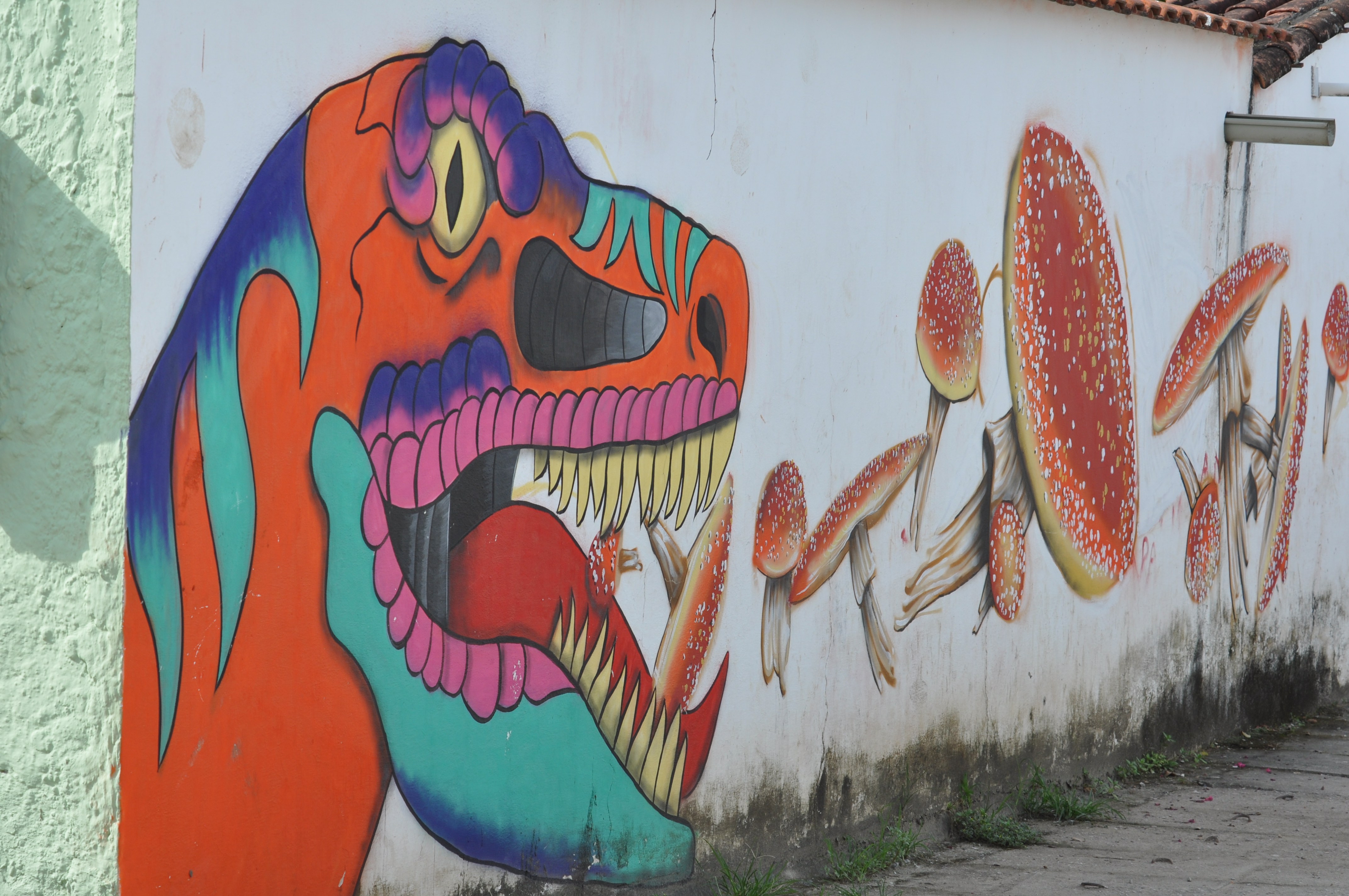This image showcases a vivid mural painted on a grimy, mold-streaked concrete wall of a building, complete with weeds and dirt creeping at its base. The mural features two distinct yet striking elements: On the left side, a brightly colored dragon's head, potentially a T-Rex or a raptor, is depicted with sharp teeth. Its predominantly orange hue is accentuated with blue and green details along the nose, while pink shades surround its mouth and yellow fangs. Facing right, the dragon's head appears poised to devour a collection of highly detailed, photorealistic Amanita muscaria mushrooms. These mushrooms feature iconic red caps adorned with white speckles and tall white stems. They seem to float at various angles, some large and others smaller, with a few even positioned inside the dragon's open mouth. Two pipes emerge from the middle of the wall, partially obscured by the artistic display, further adding to the gritty urban feel of the scene.